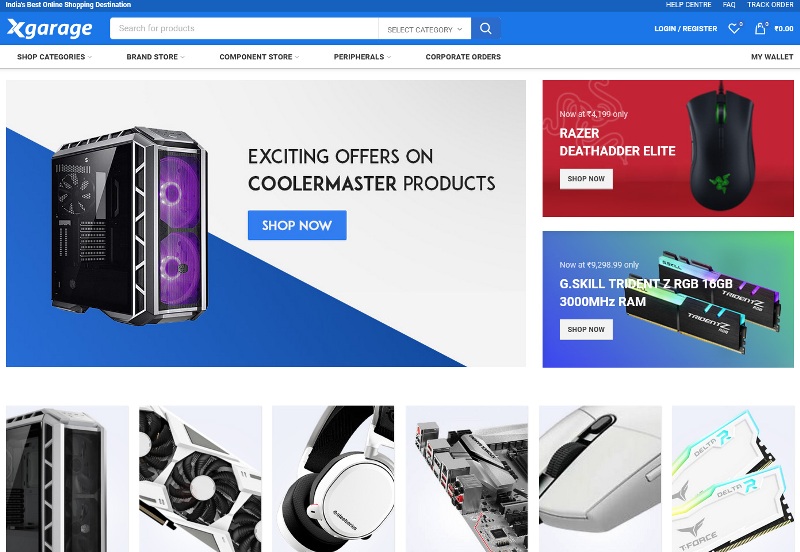The image depicts the homepage of a website called X Garage, touted as "India's best online shopping destination" displayed prominently at the top. The header features a sleek blue bar followed by a white search bar on the right. Adjacent to the search bar, options to "Log In" and "Register" are available, accompanied by a small shopping cart icon.

Directly below this header, there is a navigation menu listing: "Shop Categories," "Brand Store," "Component Store," "Peripherals," and "Corporate Orders."

The main section showcases a promotional banner featuring an image of a computer cooling tower with a caption that reads "Exciting offers on Cooler Master products. Shop Now." Beside this, an advertisement for the "Razer Death Adder Elite" mouse is displayed, highlighting the product with a black mouse image and a price tag of "₹4,199." A "Shop Now" button is prominently placed below this.

Further down, another promotional box highlights the "G.Skill Trident RGB 18GB 3000MHz RAM" with a corresponding "Shop Now" button.

Towards the bottom, several images of various electronic equipment are displayed, suggesting a diverse range of products available for purchase.